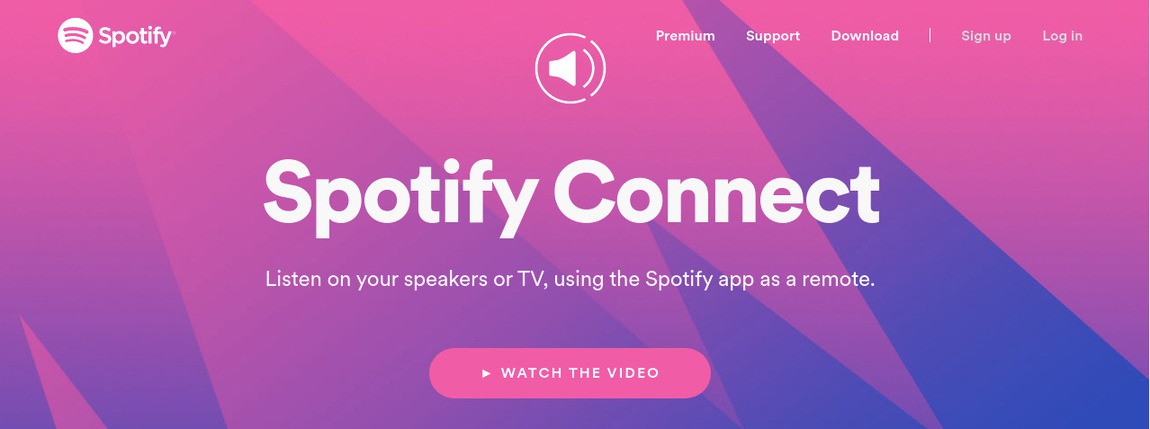Partial image of a Spotify web page featuring a vibrant banner with a magenta and purple zigzag pattern as the background. The text is in white for high contrast. 

On the left side of the banner, the Spotify logo and the word "Spotify" are prominently displayed. The center of the banner showcases a sound icon, symbolizing audio-related features. To the right of this icon are several navigation tabs, labeled "Premium," "Support," "Download," "Sign Up," and "Log In," facilitating easy access to different sections of the platform.

Below this, the banner introduces "Spotify Connect" with the subtitle, "Listen on your speakers or TV using the Spotify app as a remote." Accompanying this text is a magenta-colored button that reads "Watch the Video," complete with a play icon to guide users to further visual instructions.

This top-page banner appears to serve as either an advertisement or a prominent feature on the Spotify web page, encouraging users to explore and utilize the Spotify Connect service for enhanced audio experiences on external devices.